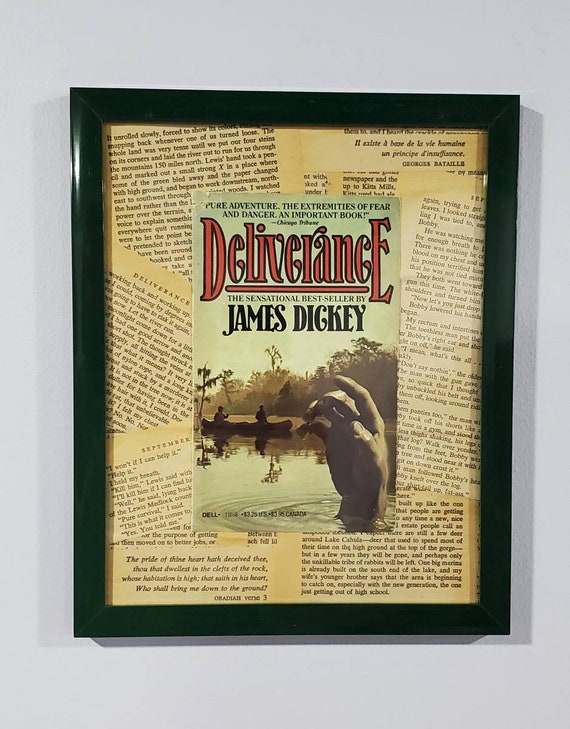This photograph captures a vertically rectangular, dark green wooden photo frame mounted on a light gray wall. The frame contains a visually striking arrangement of aged, light brown pages with black text, likely from a book. These pages, yellowed with time, surround a prominent book cover at the center. The book cover, featuring "Deliverance, the sensational bestseller by James Dickey," includes an image of a hand emerging from a water body with a boat in the background, housing two people. The scene evokes an adventurous and tense atmosphere. The detailed text on the cover reads, "Deliverance, the sensational bestseller by James Dickey," emphasizing its recognition and dramatic narrative. The shadow cast on the right-hand side of the frame adds a subtle depth to the overall image, enhancing its three-dimensional appearance.